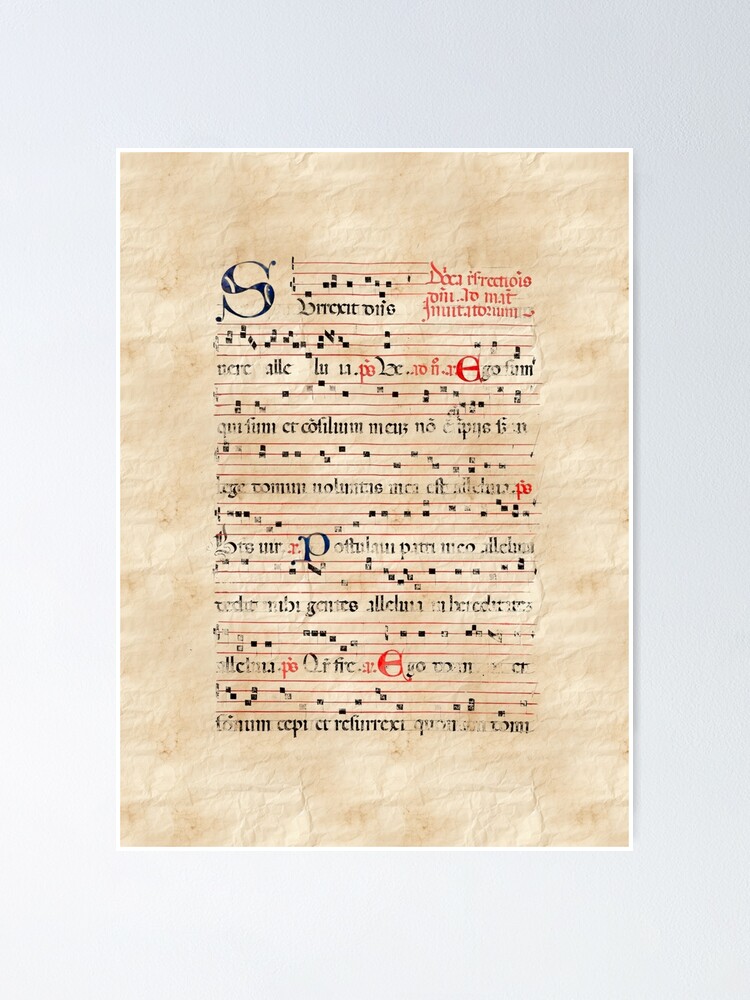The image features a framed piece of sheet music displayed digitally against a white background, creating the illusion of it hanging from a wall. The sheet music appears aged, resembling light tan, wrinkled parchment paper, and is adorned with a large capital "S" in the top left corner. The parchment contains rows of four red, horizontal lines, with black rectangular notes scattered along and between these lines. The piece also features intricate calligraphy in both black and red ink, with much of the text and annotations appearing in an undecipherable foreign language. The overall appearance is further highlighted by dark blue or very dark black ink, with red accents punctuating the content throughout.